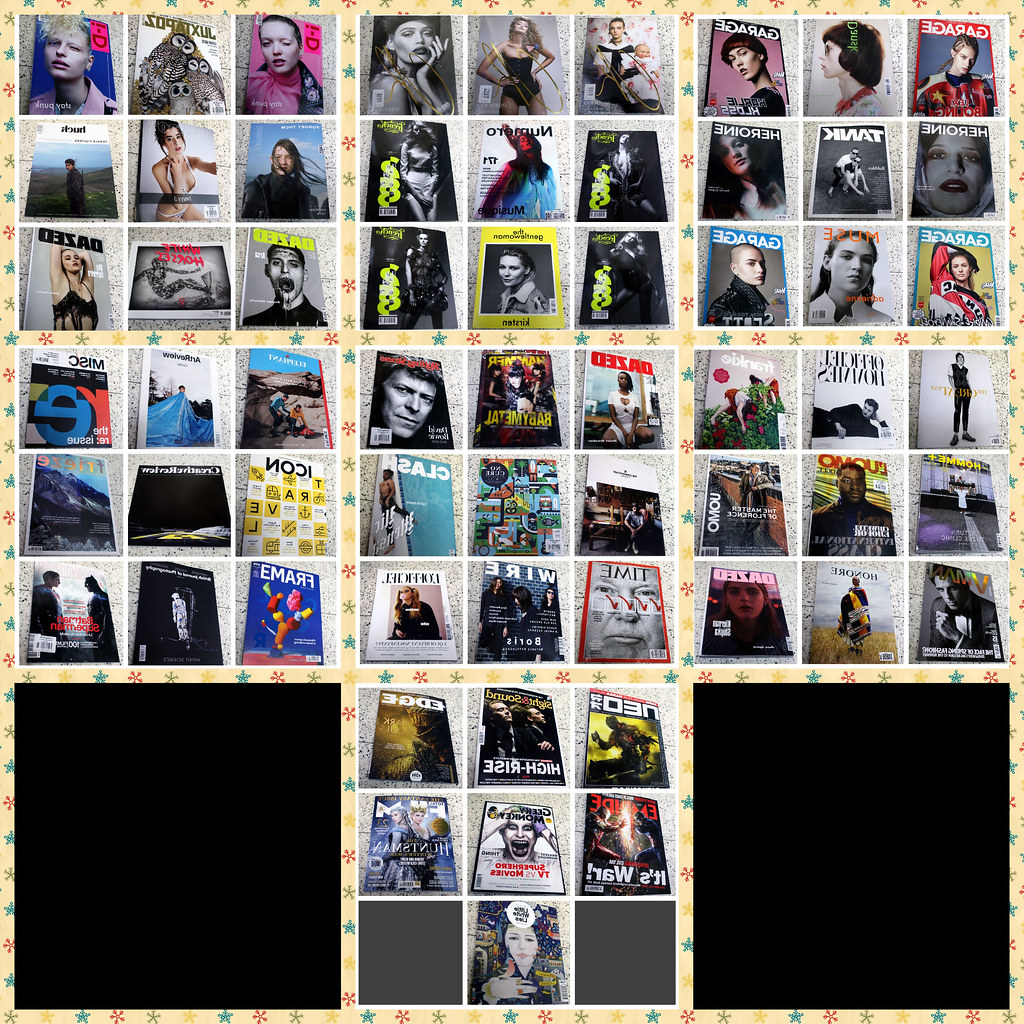The image is a detailed panorama showcasing a multitude of magazine covers arranged in a grid pattern. There are seven groups of nine covers, except for one at the bottom center which has only seven covers. Each group is organized in a three-by-three grid against a marble-like background with black spots. Two of the squares, located on the left and right sides, are entirely black. The outer edges of the collage feature a star and floral pattern starting with a green star, followed by a red flower, an olive flower, and a yellow flower. The magazine covers are diverse, displaying models in lingerie, close-up portraits, famous artists, musicians, movies, and TV shows. The grid has a bordering pattern in an off-white yellow hue with small imprints resembling snowflakes in red, yellow, and green. Some of the magazines prominently include Time Magazine, Icon Magazine, Misk Magazine, and Garage Magazine, among others, each representing various times, colors, and subjects.